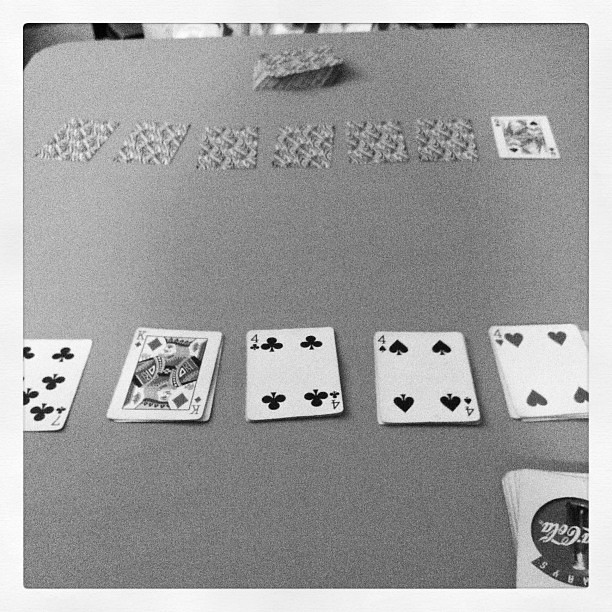A grainy black-and-white indoor photograph captures an overhead view of a tabletop filled with playing cards. In the foreground, there are five distinct piles of face-up cards: the seven of clubs, the king of diamonds, the four of clubs, the four of spades, and the four of hearts. Additionally, there is a face-down deck of cards in the lower right corner, which features a visible but inverted and backward Coca-Cola emblem on the back design.

Moving to the background, there are seven mostly face-down cards, except for one revealing the queen of spades on the far right. At the center and further back on the table, another face-down deck can be seen, having a different design from the Coca-Cola cards in the foreground.

The photograph is in focus but slightly grainy, highlighting the textures and finer details of the playing cards. The monochromatic nature emphasizes the contrast between the different elements on the table, creating a visually compelling scene dominated by the intricate patterns and randomness associated with card games.